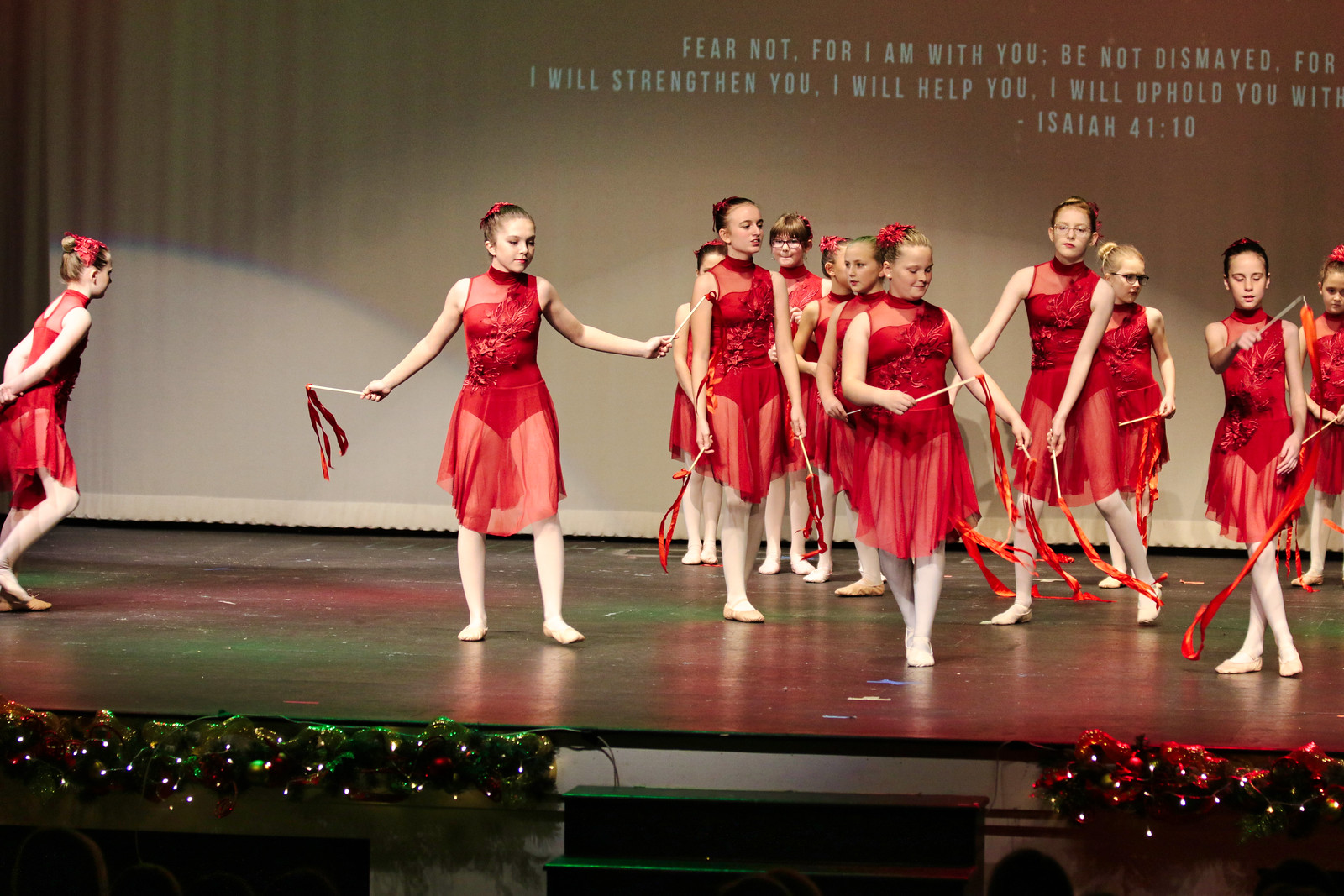The image depicts a group of middle school-aged girls on stage, dressed in coordinated red costumes reminiscent of ballerina outfits. These ensembles include a red one-piece swimsuit with a sheer, sleeveless, knee-high overlay dress and white socks or tights extending underneath. Their hair is pulled back neatly, and they each hold a stick with fabric or ribbons attached, likely used for a dance performance. Most of the girls are gathered on the right side of the stage, while one is moving from left to right. The stage is adorned with illuminated Christmas lights at the bottom, and a large projection in the background displays a Bible verse from Isaiah 41:10, which reads, "Fear not, for I am with you. Be not dismayed, for I will strengthen you. I will help you. I will uphold you with everything."